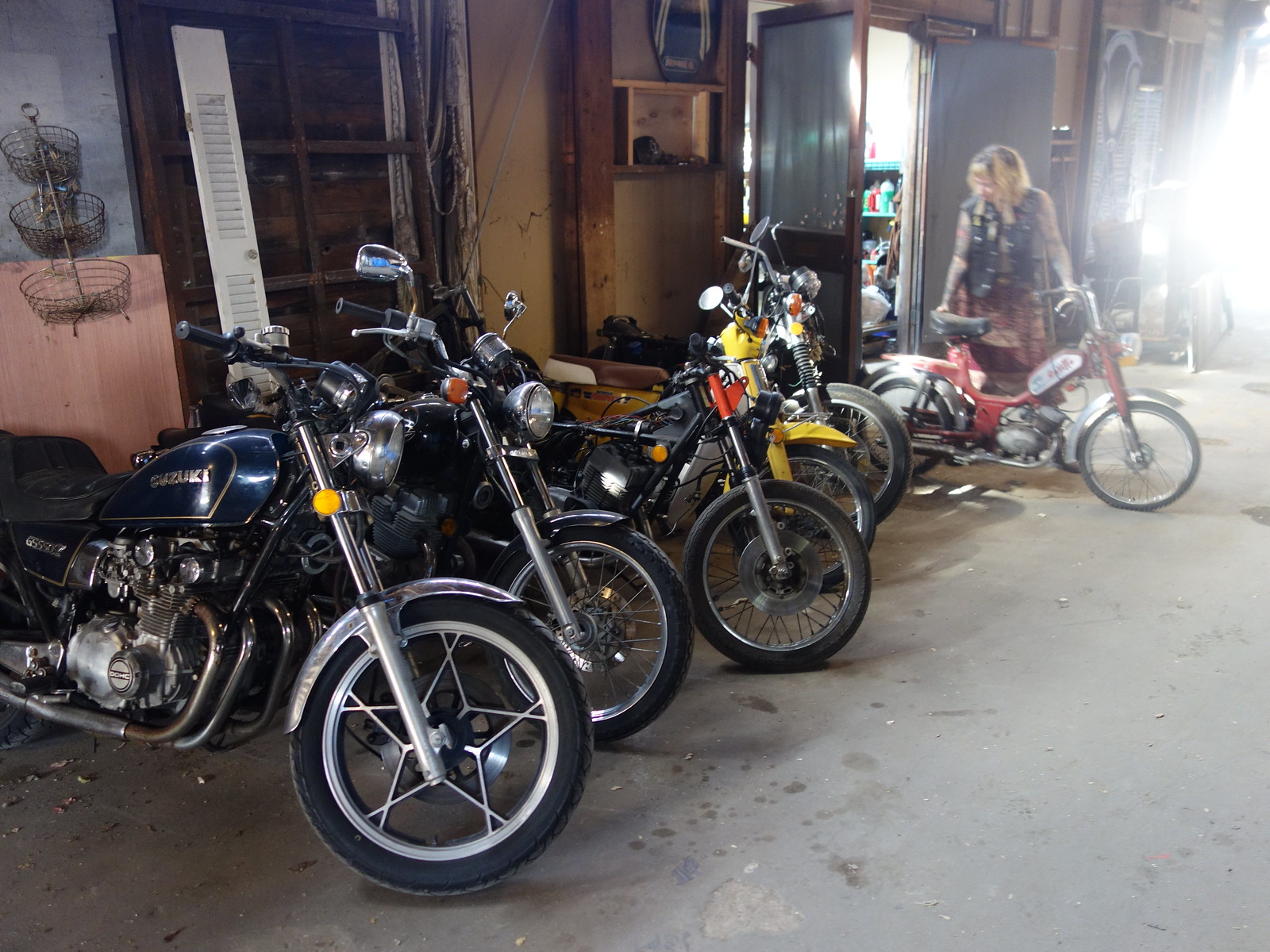In this image, we are in a spacious and somewhat cluttered garage with a gray concrete floor and tan walls. A row of six motorcycles, varying in size and type, is neatly lined up against the back wall, facing outward. Closest to the viewer is a navy blue Suzuki with its logo prominently displayed. Behind it, a larger black motorcycle with standard tires partially obscures another black bike. As the line progresses, the motorcycles decrease in size, leading up to a small red and white minibike with yellow handlebars at the far end.

A woman with blonde hair, dressed in a denim jacket over a floral skirt, is standing by the red minibike at the back of the garage. She appears to be inspecting or holding the small motorcycle, which looks custom-made, almost like a motorized bicycle. To her right, there is an open cabinet with blue bottles and various equipment visible inside. The room shows signs of being well-used, with some dirt and stray leaves scattered on the floor, and the overall atmosphere suggests it is a daytime scene as sunlight streams in. Various details, like wire baskets hanging on the wall and a pink baseboard, add to the character of this personalized and utilitarian space.